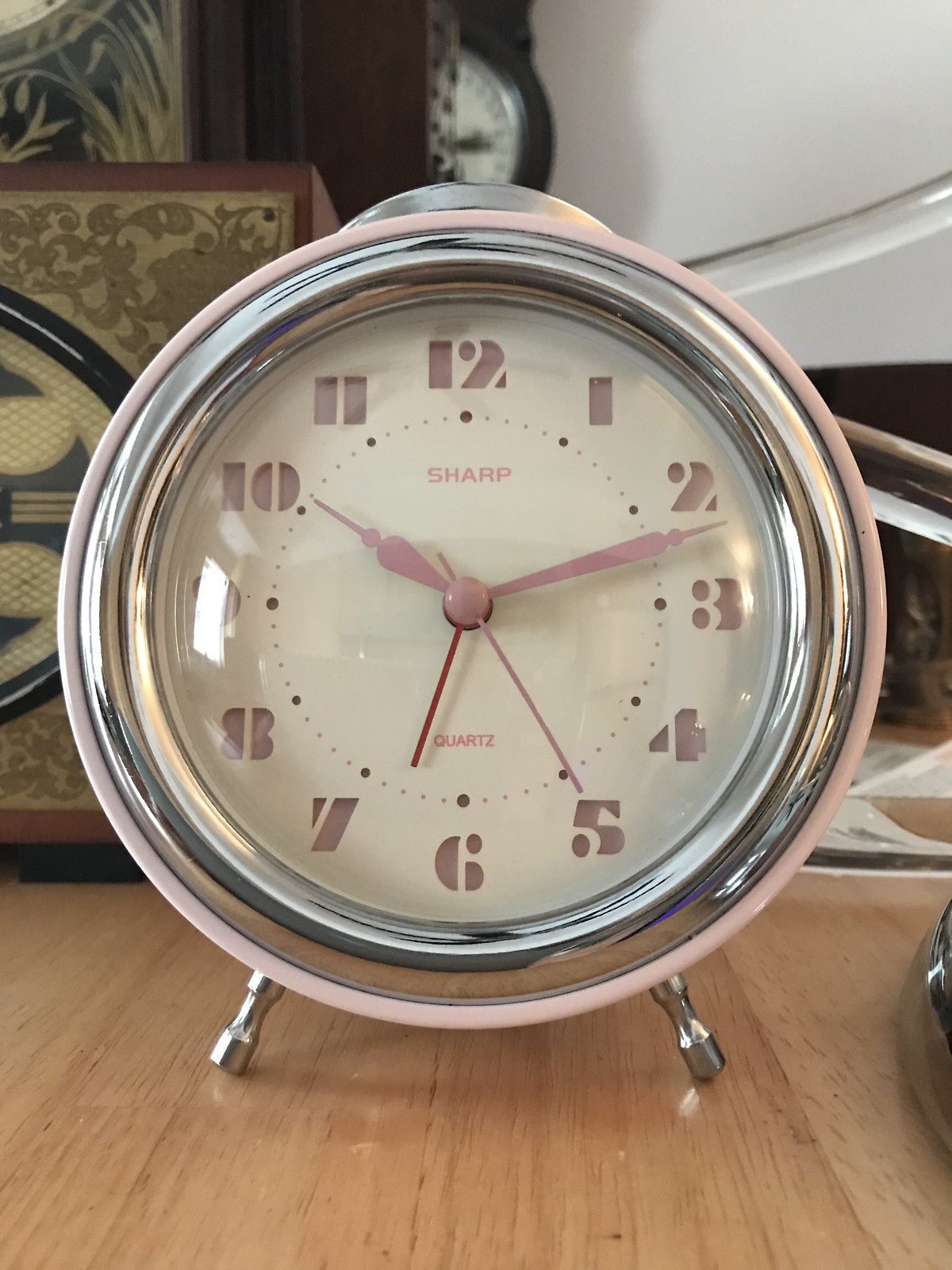The photograph captures a retro-styled Sharp quartz alarm clock positioned on a light-colored hardwood surface, likely a desk or dresser. The clock features a pastel pink body with chrome accents, including two small stainless steel legs and a chrome dome on top. Its face is enclosed by a chrome rim and has an interior that appears tan. The clock displays purple numerals from 1 to 12, with small dots indicating each minute. The hour, minute, and second hands are all pink, while an additional red hand is used for setting the alarm. The time shown is 10:12:32. Towards the bottom of the clock face, "Quartz" is printed above the numeral 6. In the background, various indistinguishable items and some wooden decorative pieces with textured patterns can be seen, along with some clear tubing.